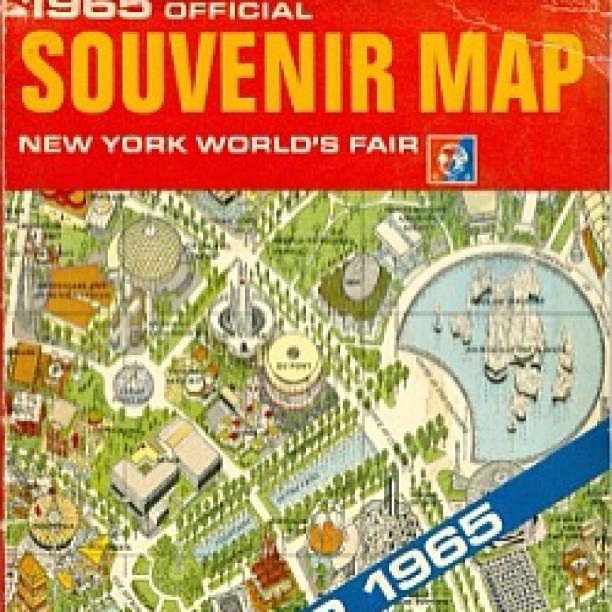The image is a large, square, and somewhat blurry cover, likely of a map or magazine from the 1965 New York World's Fair. The top part of the cover features a red rectangular background with bold, all-caps, yellow letters that read "1965 OFFICIAL SOUVENIR MAP." Beneath this, in smaller, white all-caps letters, it says "NEW YORK WORLD'S FAIR." Adjacent to this text is a red, white, and blue logo. The central portion of the image displays a detailed and colorful map, showing extensive green and white areas, domed buildings, and pathways lined with trees, giving a sense of lush landscaping. There is also a distinctive circular area on the map, likely representing water with boats, though the details are hard to make out due to the blurriness. A diagonal blue banner crosses from the middle right side to the lower middle, prominently displaying the year "1965" in bold white letters.